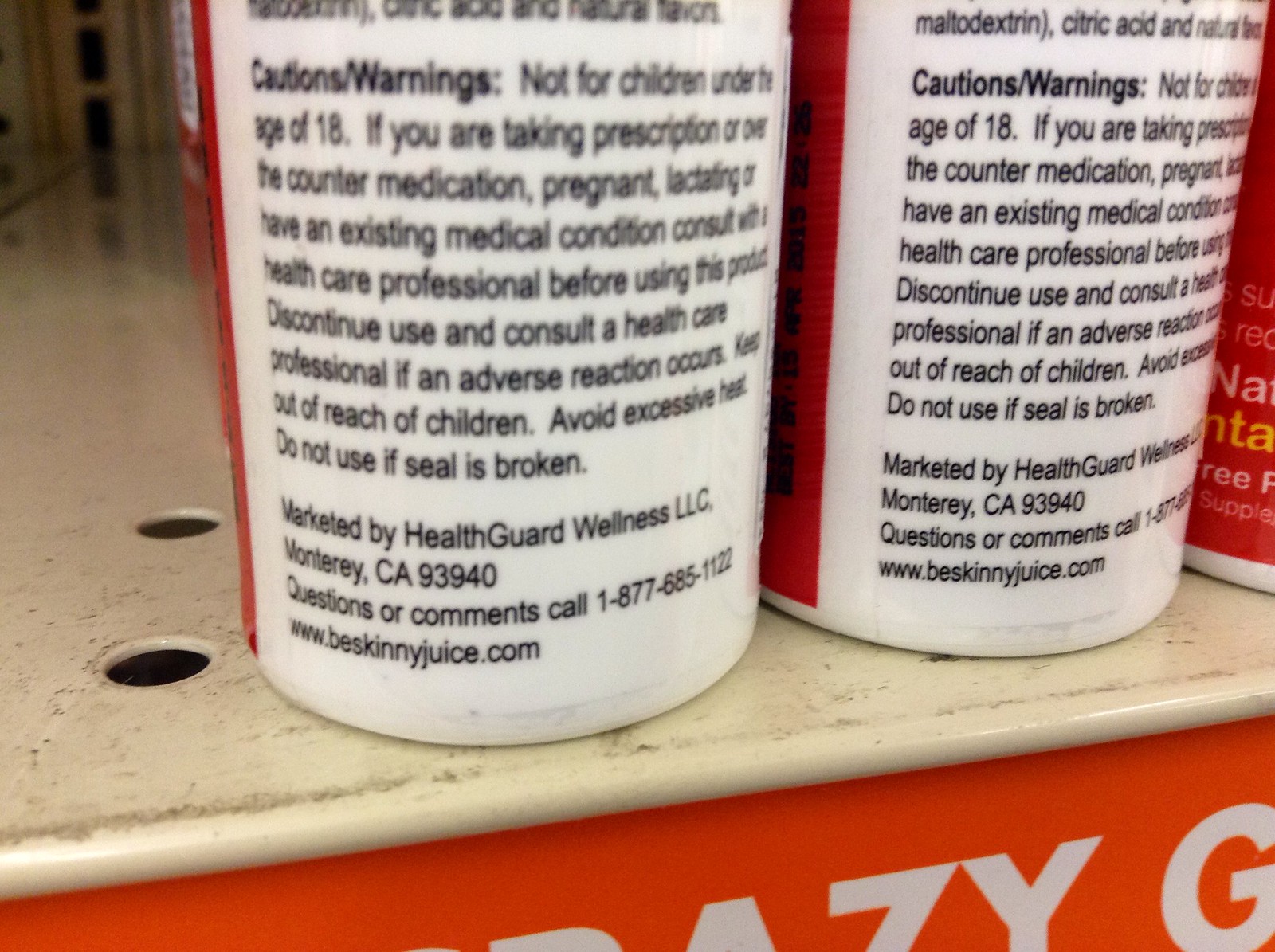A detailed close-up color photograph captures the back of two identical medication packages, specifically highlighting the dosage and caution information. The products are displayed on a white shelf, with a slight glimpse of orange on the side, possibly indicating the label or brand name area. The caution text clearly outlines that the medication is not suitable for individuals under the age of 18 and advises against use if one is taking prescription or over-the-counter medications. Additional warnings include not using the product if the seal is broken. The packaging states that the product is marketed by Health Guard Wellness, LLC, located in Monterey, California, and references a website, Biskittyjuice.com, which may be related to the product itself. The photo provides a clear view of these warnings on both packages, illustrating their identical nature and positioning on the shelf.